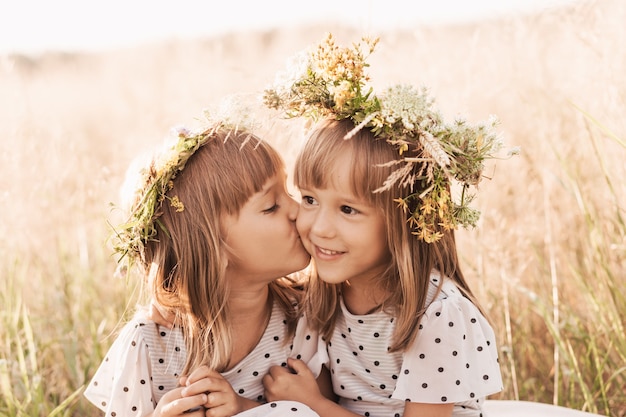This professionally taken photograph features two young girls, possibly twins or sisters, sitting in a sunlit, grassy meadow that transitions from green plants in the foreground to a blurry backdrop of beige crops, resembling tall grasses or wheat. Both girls, who are Caucasian with straight, honey-blonde hair and bangs that fall past their shoulders, are wearing white short-sleeved dresses adorned with black polka dots and faint gray stripes. They each have floral crowns made of intertwined white, beige, and yellow flowers with green leaves; the girl on the left has a slightly simpler crown compared to her sister's more elaborate one. The left girl, with her eyes closed, is sweetly kissing the smiling, open-eyed girl on the right, who looks slightly away from the camera. The image exudes a happy, serene atmosphere with its bright, sepia-toned aesthetic, highlighting the girls' tender moment amidst the sun-drenched field.